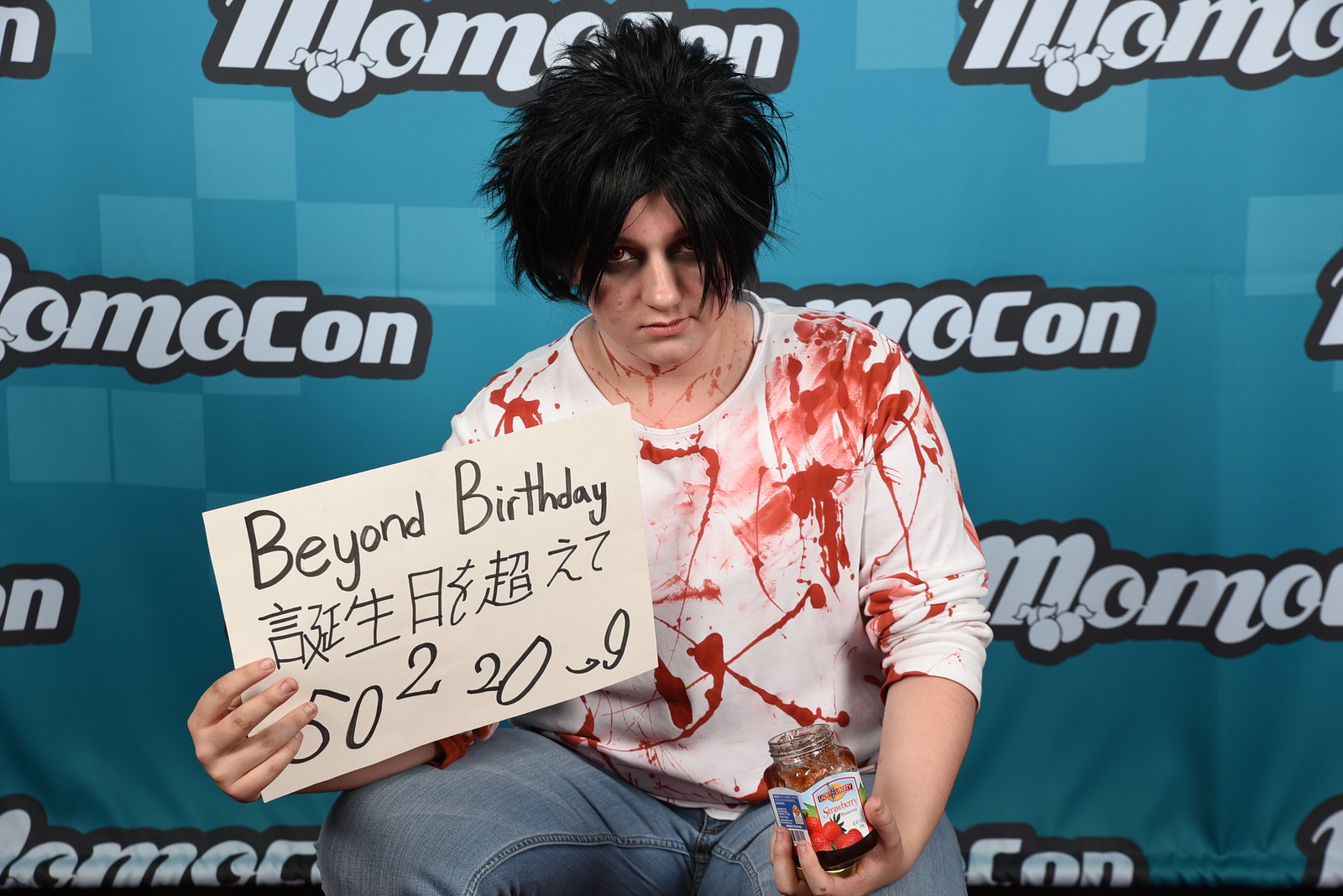In this image, a man is crouched down on his haunches, dressed in blue jeans and a long-sleeved white shirt smeared with streaks and handprints of red, resembling blood. The sleeves of his shirt are pushed up to his elbows. Red stains also cover his neck, suggesting he used the contents of the jar of strawberry preserves he's holding in his left hand to create this dramatic look. His other hand holds a white sign with black text that reads "Beyond Birthday," followed by some Asian characters and the numbers "502209." He sports a wig of thick, fluffy black hair that complements his dark, rocker-style appearance, enhanced by red contact lenses that give his eyes an eerie look. His facial expression is dark and demeaning, reminiscent of a punk band persona. The backdrop features a blue banner covered in the word "MomoCon" with geometric patterns, creating a vivid contrast that highlights his striking appearance.